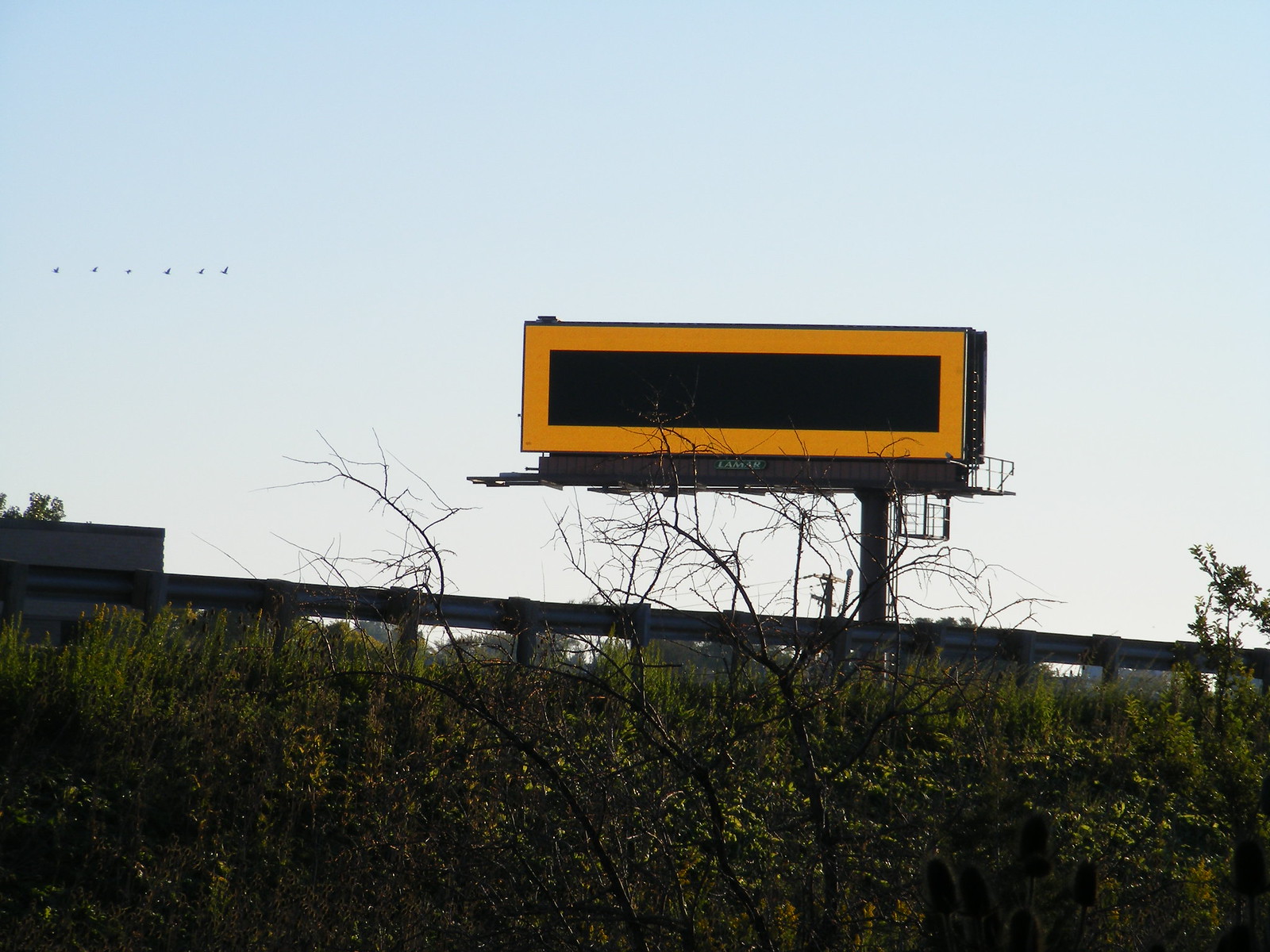The photograph captures a typical roadside scene with a significant focus on a large, unusual billboard. The billboard, prominently displayed on a single pole, features a muted orange-yellow border framing an entirely black center, suggesting it may be intended to represent the National Geographic logo or simply remains unlit. A faint line of unreadable wording, potentially "Lamar," is visible at the bottom. Below the billboard, a metal guardrail separates the foreground's green area, which is dotted with tall grasses and sparse, leafless trees. Power lines add a subtle presence in the distant background. The scene is set under a clear blue sky, punctuated by a line of six small black birds flying in a single file in the upper left corner, adding a touch of life to this otherwise still environment.